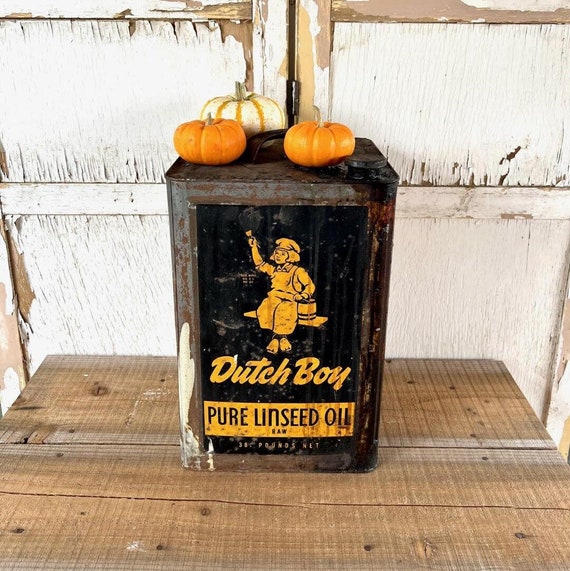The image depicts a large, rusted, and patinated metal canister prominently labeled "Dutch Boy Pure Linseed Oil, Raw." The label features a vintage design in black or navy, with a golden-yellow image of a child sitting on a ledge, holding a paintbrush in one hand and a paint bucket in the other. The canister, which is estimated to weigh several pounds, sits on a worn wooden platform amidst a rustic setting. Adorning the top of the canister are three small pumpkins: two are traditional orange, while the larger one is predominantly white with orange accents. The background consists of a weathered, white-painted wooden wall with peeling paint, suggestive of an old barn or shed.